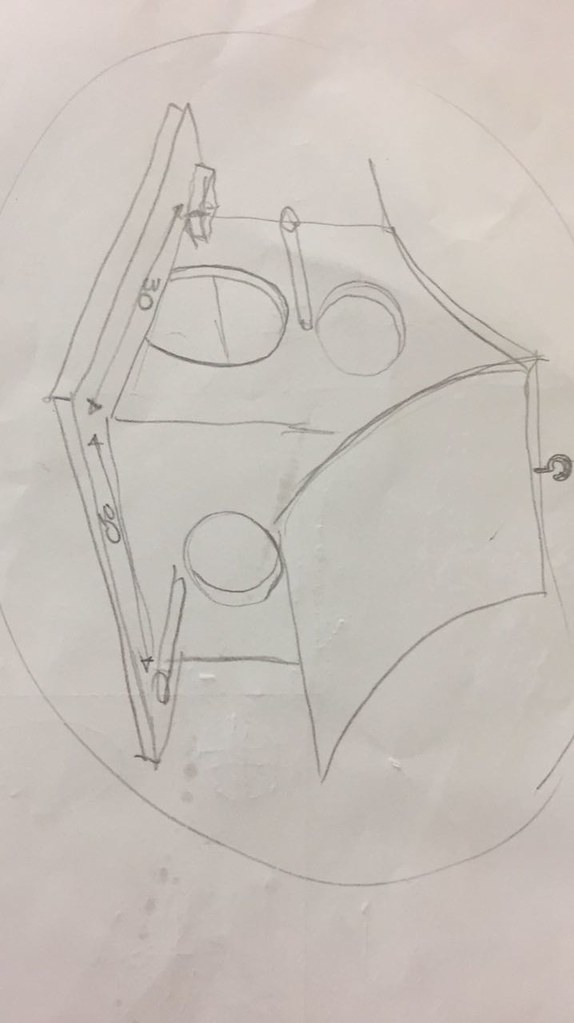On a sheet of white paper, there's a meticulously drawn circle that frames a pencil sketch of a birdhouse. The birdhouse is illustrated with a sloping, concave roof, topped by a definitive edge that supports a dark gray hook for hanging. The intricate roof design showcases its two concave sides joining seamlessly at the top where the hook is situated.

The side of the birdhouse features a circular entrance hole accompanied by a small ledge beneath it. Notably, the dimensional aspect of the drawing reveals the interior space of the birdhouse, allowing a glimpse inside the top window and front door. Measurements marked with the number "30" are visible on both the side and front, suggesting dimensions or a design reference.

Additionally, at the front of the birdhouse, there is a small box placed just outside the entrance, adding to the intricate details. Surrounding the birdhouse is a ledge approximately an inch and a half wide. The platform on which the birdhouse stands appears to be about half an inch thick, providing a solid base for the structure.